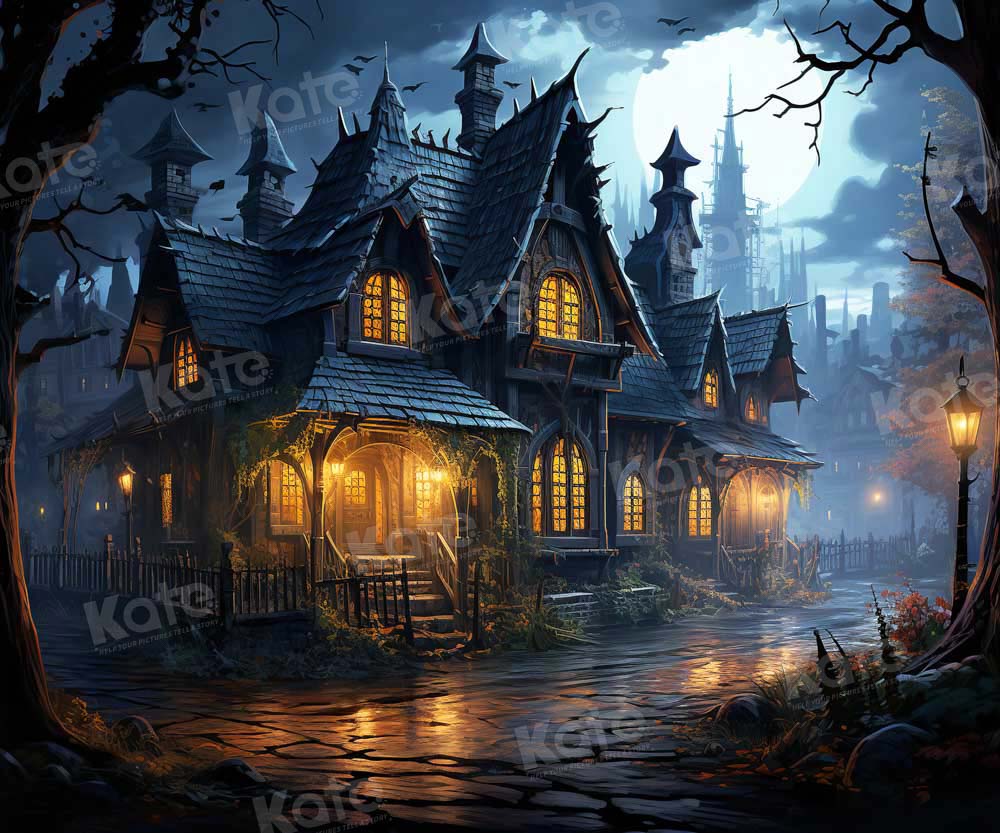The image depicts a dark, slightly rickety house with various funky spires and turrets on the roof, complemented by cedar shake shingles. Its eerie atmosphere is accentuated by the house's illumination with warm amber lights glowing through the arched windows and entryway, casting an inviting yet mysterious glow on the cobblestone path leading to the door, which is further illuminated by amber street lanterns. Framed by large trees, the scene is set at nighttime under a full, bright moon partially obscured by clouds. There are crows perched on the roof and flying overhead, adding to the unsettling ambiance. The house might belong to someone malevolent or a witch, reminiscent of an abode from the Addams Family. In the distant background, castles and spires are faintly visible, enhancing the image's gothic charm. Watermarks reading "KATE" are scattered across the image, with smaller, illegible text beneath them.